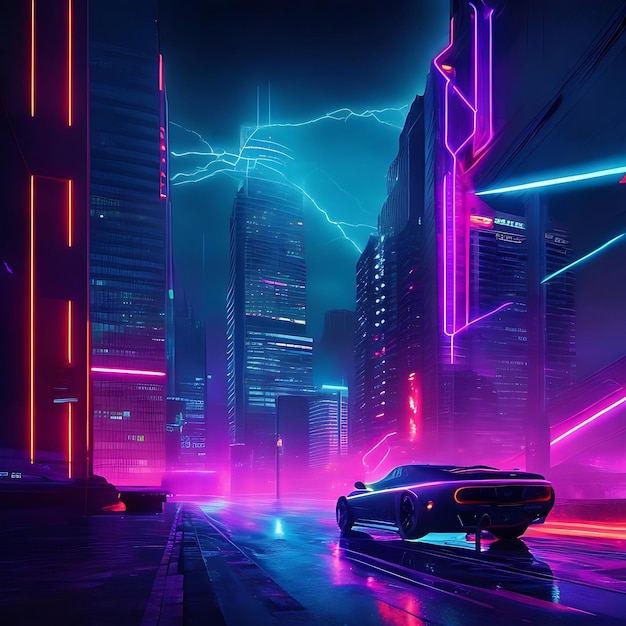This digital artwork portrays a cyberpunk cityscape at night, vividly illuminated with a mesmerizing amalgamation of neon colors. The bustling city is dominated by towering skyscrapers bathed in bright neon lights, predominantly in hues of pink, blue, and orange. These lights cast an otherworldly glow across the scene, accentuating the futuristic aesthetic.

In the foreground, a purple sports car races along a multicolored street, predominantly tinged with shades of purple and pink. The road glistens as if damp, further enhancing the visual depth and atmosphere of the image. The car, viewed from the rear, appears somewhat distorted and not quite grounded, hinting at the AI-generated nature of the artwork.

Surrounding the street are sidewalks, while the mid-ground is filled with soaring buildings that seem to blend seamlessly into each other, reflecting a surrealistic design. Among the buildings, a particularly tall skyscraper stands out, adorned with antenna towers and crisscrossed by striking teal-green lightning bolts against a darkened sky.

This piece exudes a strong cyberpunk and synthwave vibe, capturing the neon-lit essence of a digital cityscape rendered with both creativity and structural anomalies.